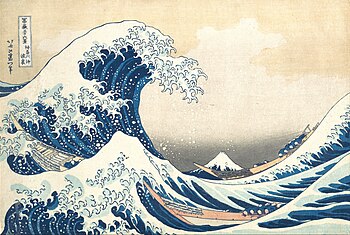This image captures the iconic Japanese painting, "The Great Wave off Kanagawa," by the renowned artist Katsushika Hokusai. The composition beautifully illustrates the powerful movement of immense, curling waves rendered in striking blue hues, with distinct, solid white foamy crests. Despite the simplicity of the style, an abundance of intricate details can be observed, such as three or four small boats caught in the tumultuous sea. A massive wave on the left dwarfs the others, embodying the drama and energy of the scene. Over the horizon, a diminutive, snow-capped Mount Fuji provides a stark contrast against the tumultuous sea. The sky is colored in a muted beige or tan, enhancing the overall tranquility and balance of the composition. In the corner of the painting, Japanese script can be seen, likely depicting the title and artist's signature, although the specific characters are indiscernible without knowledge of the language.